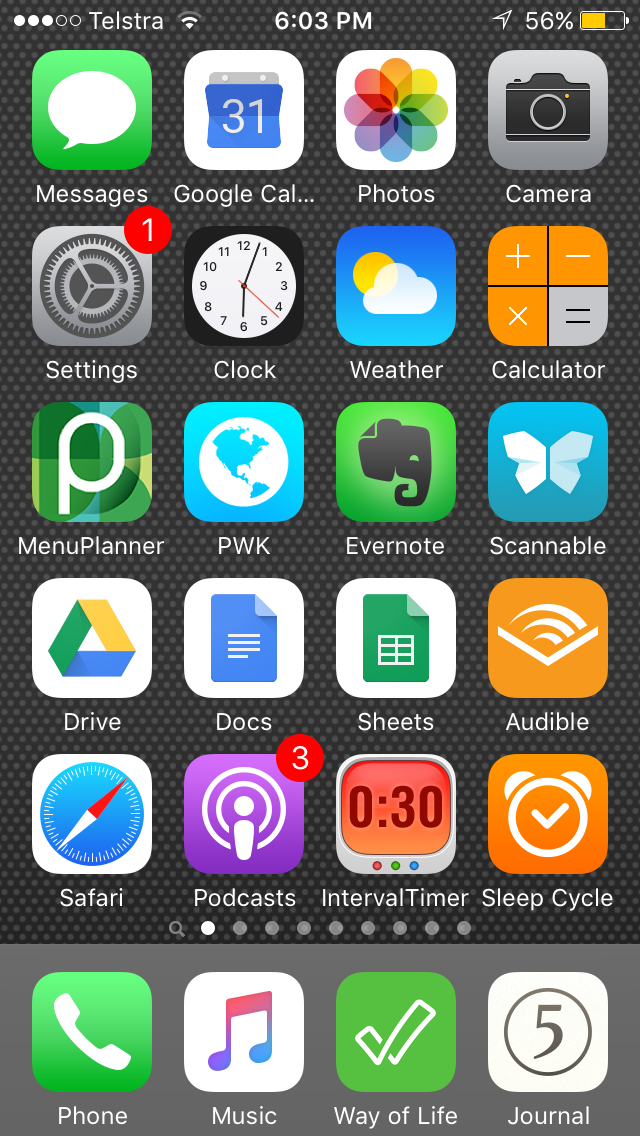The image showcases the front page of a cell phone's home screen, prominently displaying various app icons against a black background. The phone, connected to Telstra network, is currently at 56% battery level and the time is 6:03 p.m. 

The visible app icons include Messages, Google Calendar, Photos, Camera, and Settings. Notably, there is a red circle with a white '1' indicating a notification related to settings. Other displayed apps encompass a clock, weather, calculator, menu planner, PWK, Evernote, Scannable, Google Drive, Docs, Sheets, Audible, Safari, and Podcasts, with a red circle containing a '3' indicating an unread notification. Additionally, icons for Interval Timer and Sleep Cycle are seen.

At the bottom of the screen, icons for Phone, Music, Way of Life, and Journal are positioned against a gray color gradient, contrasting with the predominantly black background. This meticulous layout on the front page offers a clear and organized view of essential applications, punctuated by notifications and system alerts.